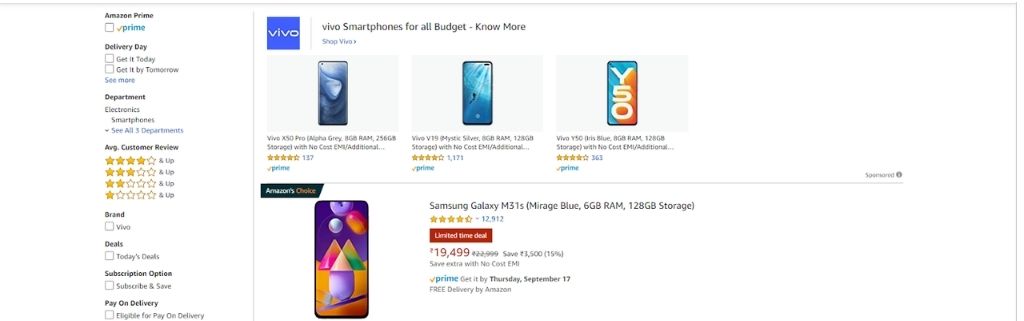This is a highly detailed screenshot from the Amazon website, featuring a selection of smartphones. On the left side, a vertical menu lists various navigation options including Amazon Prime services, delivery options like "get it today" and "get it by tomorrow", different departments including electronics and smartphones, customer review filters ranging from one to four stars, and brand options such as Vivo. Other options shown are deals like today's deals, subscription services, and payment methods including "subscribe and save" and "pay on delivery".

On the right side of the screenshot, a blue square prominently displays the Vivo brand logo in lowercase white letters with the caption, "Vivo smartphones for all budget. Shop Vivo." Below this, there are detailed listings of three smartphones from Vivo:
1. **Vivo X50 Pro** in Alpha Gray, featuring 8GB RAM and 256GB storage. This phone is highlighted with 4.5 stars based on 137 ratings and mentions "no cost/EMI additional".
2. **Vivo V9** in Mystic Silver, offering 8GB RAM and 128GB storage with 4 stars from 1,171 ratings, similarly indicated with "no cost/EMI additional".
3. **Vivo Y50** in Iris Blue, also providing 8GB RAM and 128GB storage, rated at 4 stars from 363 ratings and noted with "no cost/EMI additional".

In addition, there is a featured model with an "Amazon's Choice" banner: the **Samsung Galaxy M31s** in Mirage Blue. This smartphone displays a vibrant geometric design primarily in purple and orange tones. It comes with 6GB RAM and 128GB storage. It has been highly rated at 4.5 stars from 12,912 ratings and is available as a limited time deal priced at $19,499, marked down from $22,999 with a savings of $3,500, representing 15% off. The listing also highlights additional savings options with "no cost EMI" and Prime benefits, including guaranteed delivery by Thursday, September 17th, and free delivery by Amazon.